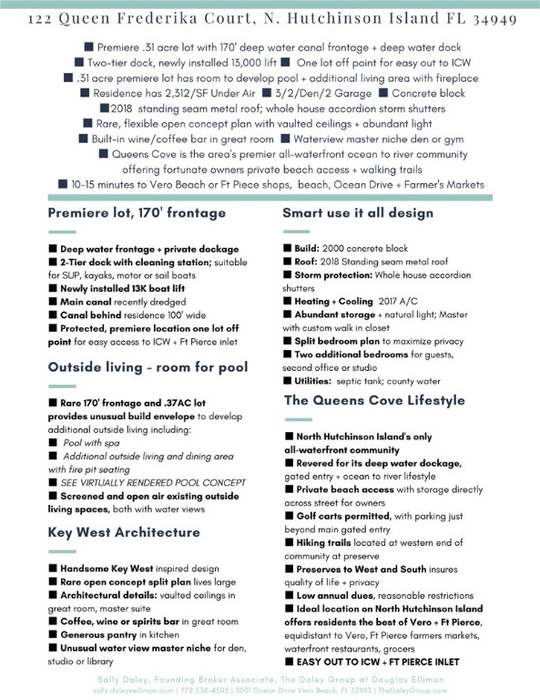A detailed real estate advertisement is presented on a white background, beginning with the address "122 Queen Frederica Court, North Hutchinson Island, Florida, 34949" prominently written at the top. The text is organized with square bullets in black and separated by turquoise bars. The focal point is a premier 0.31-acre lot featuring 170 feet of deep water canal frontage and a deep water dock. Additional amenities include a two-tiered dock, a flexible open-concept plan, a built-in wine and coffee bar in the great room, and master suites with water views.

The advertisement is structured into several sections, each detailing different features. In the left column, it mentions a Premier Lot with 170-foot frontage, outlining seven key features. Below it, "Outside Living" suggests there is room for a pool and lists five features. Toward the middle, phrases such as "Key West Architecture," "Smart Use All Design," and specific details like "Built in 2000 with concrete block construction," "Roof updated in 2018," and "Golf carts permitted," are highlighted with bullet points.

The right column features "Queens Cove Lifestyle," supported by eight bullet points, emphasizing the lifestyle benefits of the development, such as "easy access to ICW" and "Fort Pierce Inlet."

Overall, the document is a comprehensive property description, catering to potential buyers interested in upscale, waterfront real estate with plentiful amenities and thoughtful design details.